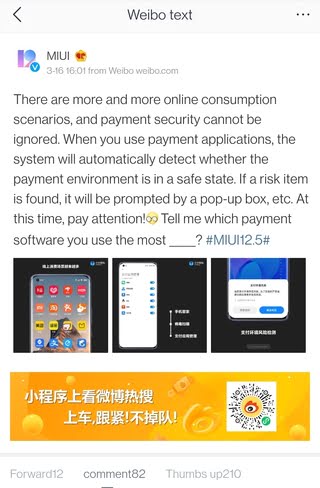This image appears to be a screenshot of a smartphone displaying a Weibo post. 

In the upper-left corner, there is a small left-pointing arrow. Centered at the top is the text "Weibo," and in the upper-right corner are three vertically aligned dots, indicating additional options. Just below this, there is a small icon with a check mark or possibly the letter "V," followed by "MIUI" in all capital letters. The timestamp reads "316, 16.01 from Weibo.com."

The post discusses the increasing number of online consumption scenarios and the importance of payment security. It mentions that when using payment applications, the system will automatically assess whether the environment is safe, triggering a pop-up warning if any risks are detected. The post advises users to pay attention to these warnings. Accompanying the text is an icon of a yellow face wearing glasses, asking, "Tell me which payment software you use the most." This is followed by hashtags "#MIUI 12.5."

At the bottom of the screen, there are three smaller images against black backgrounds. The first image shows a smartphone screen with various icons, the second image is a blurry full-screen shot of a smartphone, making specific details hard to discern, and the final image shows the bottom part of a smartphone screen, also with blurry text. Beneath these images is a yellowish-orange banner with text in a foreign language.

The post concludes with three interaction metrics at the very bottom: "Forward 12," "Comment 82," and "Thumbs up 210."